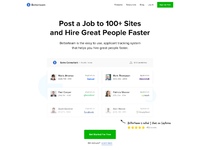This image, though blurry, appears to be a promotional banner for an applicant tracking system called Better Team. Central to the image is the Better Team logo, accompanied by a green sign that reads "Get Started." The main slogan prominently displayed on the banner states, "Post a job to 100 sites and hire great people faster." Below this, the text emphasizes the convenience and efficacy of the service with a line that reads, "Better Team is the easy to use applicant tracking system that helps you hire great people."

Though the image's low resolution makes it difficult to read the finer details, several bullet points and smaller text sections can be discerned around the banner. Moreover, a noticeable five-star rating is highlighted by an arrow, underscoring user satisfaction. The image also indicates where users can get started with the service or log in if they are already members. Despite its quality, the banner aims to attract those looking to streamline their hiring process via Better Team's reputed platform.